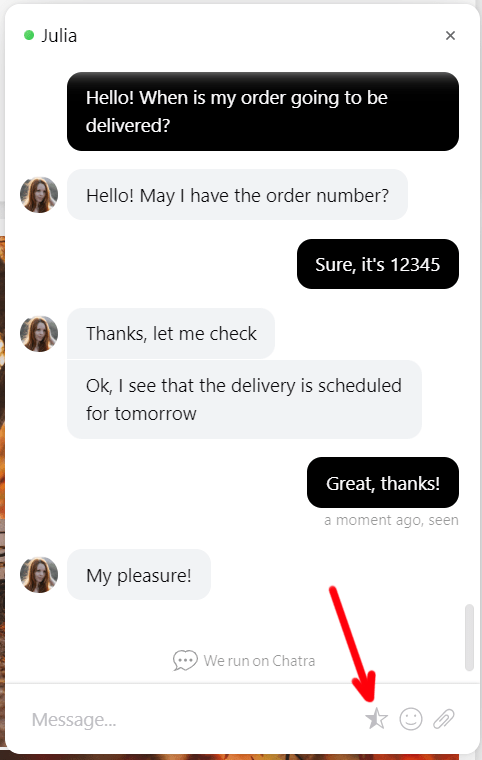Screenshot of a text conversation within a chat application. The chat window is a white box bordered by a gray outline. At the top of the window, a green circle with the name "Julia" indicates the active chat participant, accompanied by an "X" button on the top right for closing the chat.

The conversation itself starts with a black text box from the user that reads, "Hello, when is my order going to be delivered?" Below this, a light gray text box shows a reply from Julia, whose profile picture is a woman with red hair. Julia's response is, "Hello, may I have the order number?"

Following Julia's message, another black text box from the user states, "Sure, it's 1-2-3-4-5." Julia then responds in another gray text box saying, "Thanks, let me check." After a brief check, Julia updates, "Okay, I can see that the delivery is scheduled for tomorrow." 

The user follows up with a final black text box saying, "Great, thanks." with a time-stamp "a moment ago" and the status "seen." Julia completes the conversation with a gray text box saying, "My pleasure. We run on Chitra."

At the bottom right corner of the chat window are icons for additional actions: a star icon with a red arrow pointing at it, a paperclip icon, and a smiley face icon.